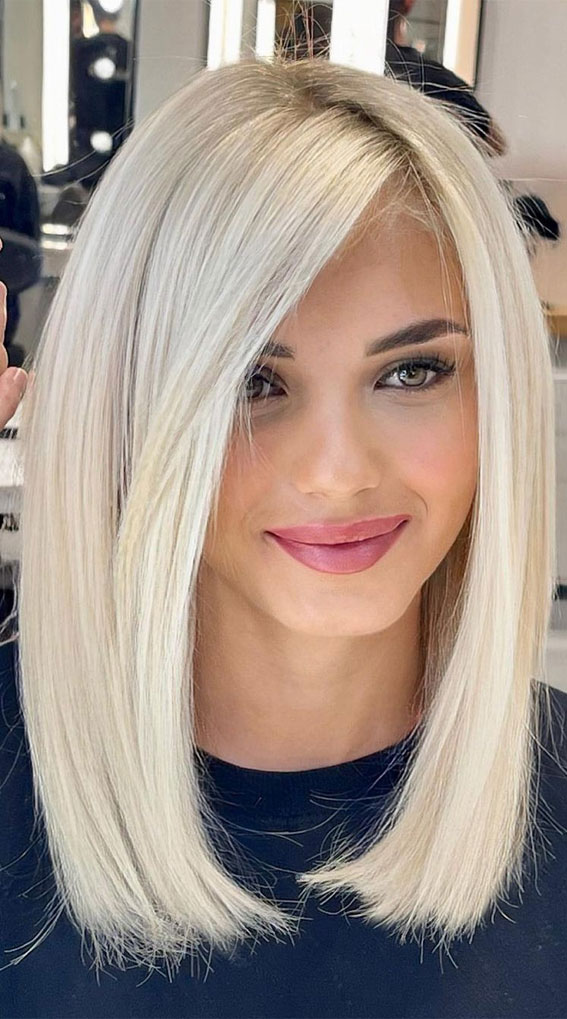A beautifully detailed photo captures a young Caucasian woman seated in a hair salon, elegantly modeling her new hairstyle. She has striking dark, manicured eyebrows and mesmerizing greenish-gray eyes that complement her radiant complexion. Her long, platinum blonde hair is meticulously styled; it is parted slightly off-center, draping gracefully around her face and angled with precision, almost like bangs subtly covering part of her eye and cascading down to her chest. She wears a smile that adds to her serene and poised appearance, accentuated by the red lip gloss she wears. Draped over her torso is a dark blue cover typically used in salons. The background reveals a bustling salon environment, with reflections of mirrors, side lights, a hairdryer, utensils, and subdued figures of hair artists attending to clients. This scene, likely intended for a hairstyle portfolio, is a harmonious blend of beauty, style, and professional craftsmanship.